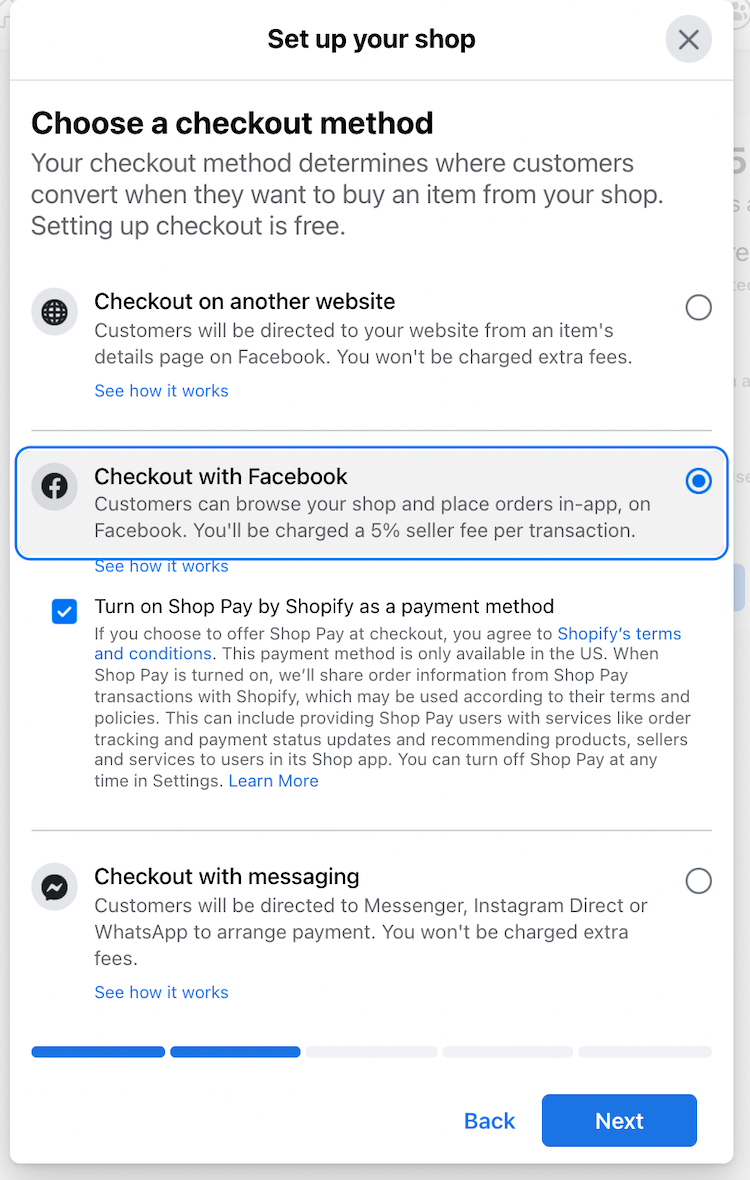The image displays a web page designed for setting up an online shop. Centered at the top of the page, a header reads "Set Up Your Shop." The page features a clean design with a white background and blue accents used for buttons and highlights around sections. The main body text is predominantly black.

Directly below the header, the text prompts the user to "Choose a Checkout Method," explaining that this choice determines where customers complete their purchases. Various checkout options are provided, such as:

- **Check out on another website:** A selectable option.
- **Check out with Facebook:** Also selectable, and currently chosen, as indicated by a tick mark within a circular checkbox.
- **Turn on Shop Pay by Shopify:** Presented as an alternative payment method.
- **Check out with Messaging:** Described in detail at the bottom of the page.

The bottom section elaborates that "Check out with Messaging" allows customers to use Messenger, Instagram Direct, or WhatsApp to arrange payments, although extra fees apply. A link labeled "See how it works" provides additional information.

Navigation buttons labeled "Back" and "Next" are positioned at the bottom of the page, enabling the user to move to the previous screen or proceed to the next step.